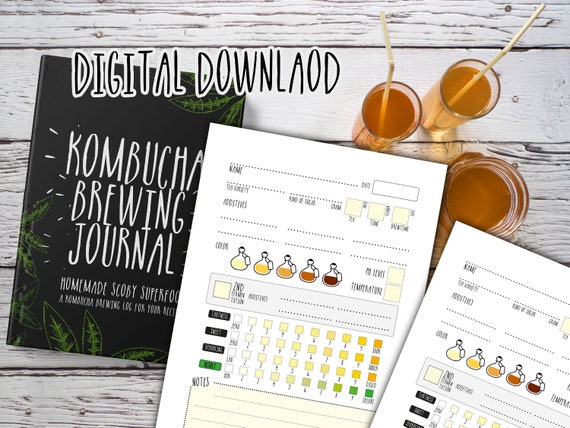This image is a detailed social media advertisement for a digital download of a "Kombucha Brewing Journal" e-book. The scene is set against a whitewashed wooden background with an overhead view. Central to the image is a black journal featuring white lettering that reads "Kombucha Brewing Journal, Homemade, Scobie Superfood." The cover also has small white text beneath the main title, though it's challenging to read all of it clearly.

Accompanying the journal are two preview pages showcasing the journal’s internal layout. These pages display a brewing log where users can document the type of kombucha, brewing date, color, pH levels, and any additional notes. The pages contain various colored boxes and blank sections to fill out brewing details.

In the top right corner of the image, three glasses filled with light brown kombucha are visible. Two of the glasses have straws, and there is also a jar of kombucha next to them. The glasses and jar add a practical touch, visually connecting the journal to the kombucha brewing process.

Noteworthy is the digital download notice at the top left of the image, aimed at potential buyers, and a typing error where "download" is misspelled as "DONWLOAD." The overall layout and elements presented in the image suggest it is a visually appealing advertisement aimed at kombucha enthusiasts, encouraging them to purchase the downloadable brewing journal, possibly on platforms like Etsy.